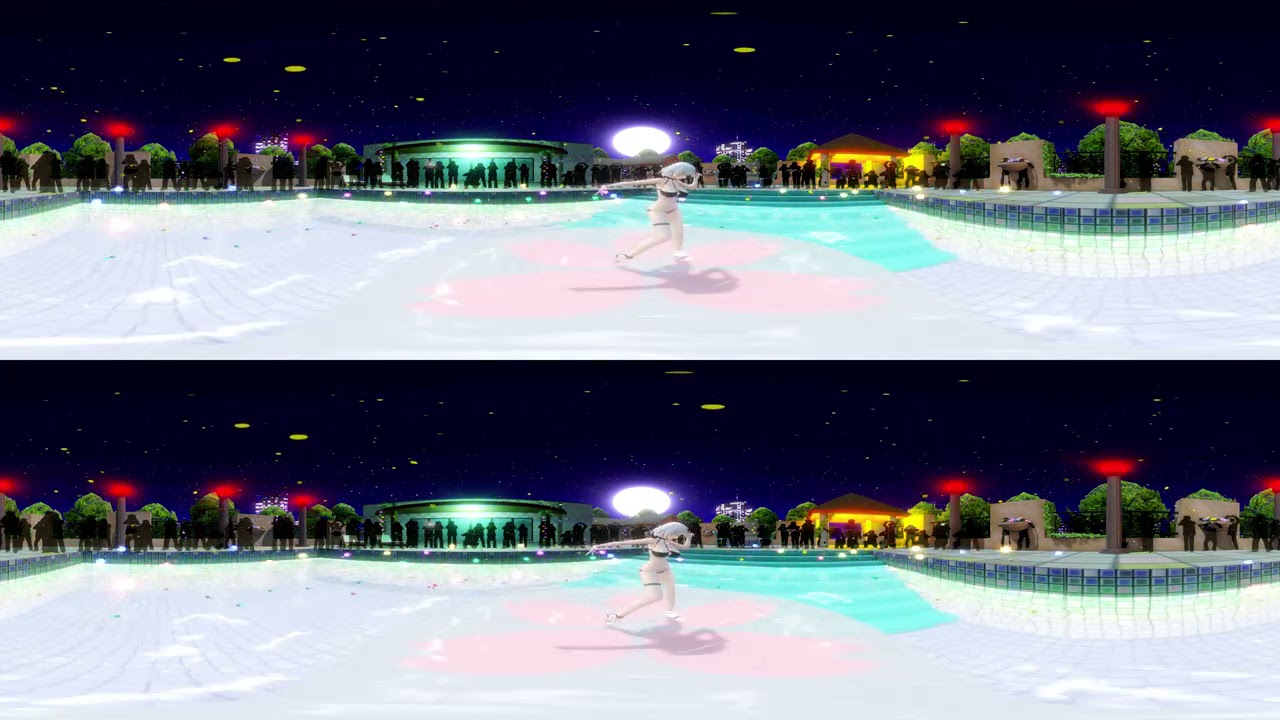The image comprises two horizontally aligned, identical digital art scenes stacked on top of each other. Each scene features a cartoonish female character with white skin, wearing a bikini-like outfit and white hair, standing in the center, appearing to dance. Behind her is a pool surrounded by silhouetted figures who seem to be either watching or dancing. The ground surface resembles ice or an icy environment. In the background, there are yellow structures with roofs, trees, and multiple lampposts topped with red lights. The dark blue sky, adorned with white stars and the moon, enhances the nighttime outdoor setting. Additional elements include a set of stairs leading down to the icy ground and possibly, oval-shaped yellow objects reminiscent of flying saucers in the sky.